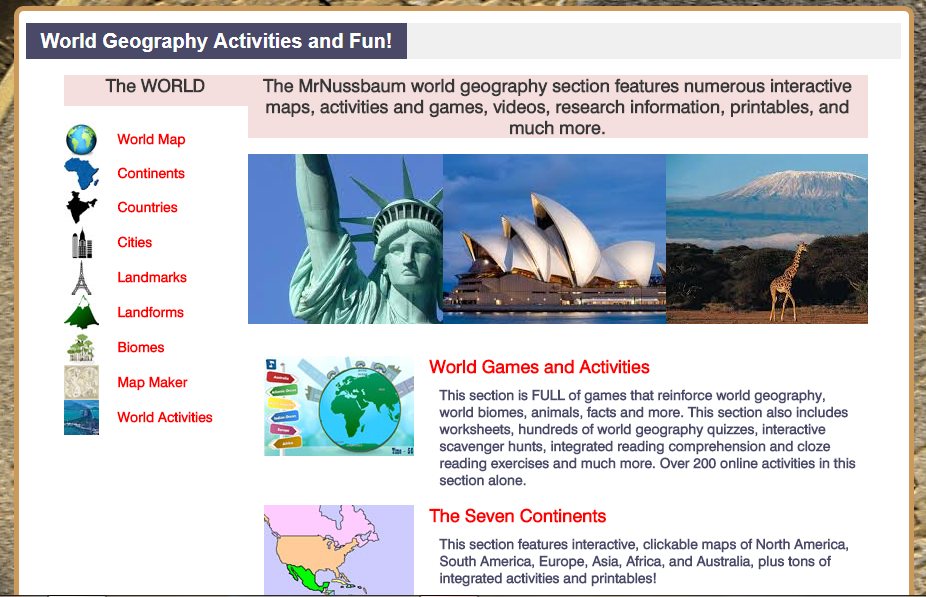This is a detailed caption for the image you described:

---

This image is a vibrant screenshot of a website with a white background. Dominating the top portion of the screen is a large, dark rectangle featuring the title "World Geography Activities and Fun" in bold white letters. Below this header, a soft purplish-red background appears, with black text that reads, "The World." The text elaborates, stating: "The Mr. Nussbaum World Geography section features numerous interactive maps, activities, and games, videos, research information, printables, and much more."

On the left side of the screen, beneath "The World," a white section displays various icons and accompanying text in red. From top to bottom, the icons include:
- A globe labeled "World Map"
- A continent icon labeled "Continent"
- A country icon labeled "Countries"
- Various images including buildings, cities, the Eiffel Tower 
- A mountain icon possibly representing "landforms"
- Trees symbolizing "biomes"
- A map icon labeled "Map Maker"
- A blue object labeled "World Activities"

Central to the right of the main body is a colorful collage featuring the Statue of Liberty, the Sydney Opera House, and a giraffe under what appears to be Mount Kilimanjaro. Below this collage, a text section with a globe icon reads, "World Games and Activities." It highlights that this area is packed with games that reinforce knowledge of world geography, biomes, animals, and facts, as well as worksheets, hundreds of world geography quizzes, interactive scavenger hunts, integrated reading comprehension, COLZE reading exercises, and over 200 online activities.

Towards the bottom, a bright, colorful image depicting the Americas is accompanied by the text "The Seven Continents." This section offers interactive clickable maps of North America, South America, Europe, Asia, Africa, and Australia, along with numerous integrated activities and printables.

---

This extensive caption captures all the prominent elements and details of the website screenshot.